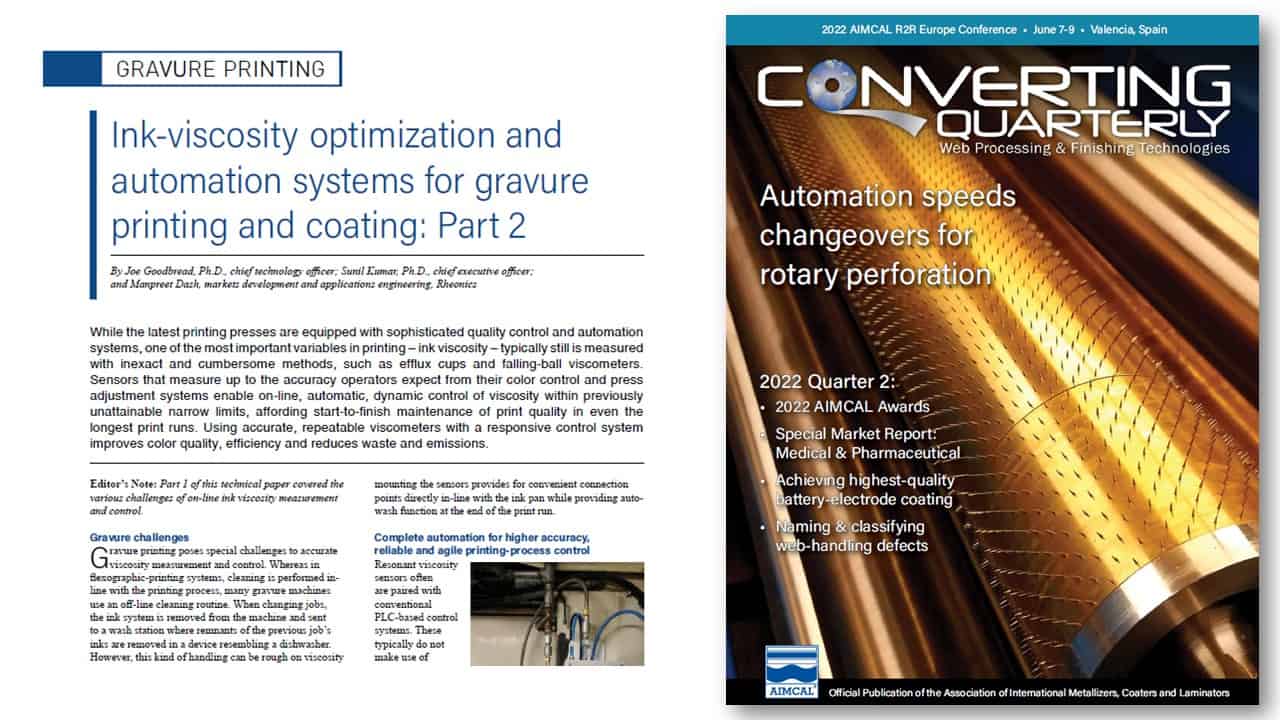This image depicts a detailed photograph of a magazine spread. The right side showcases the cover of "Converting Quarterly," a publication focused on web processing and finishing technologies. The cover highlights the 2022 AIMCAL R2R Europe Conference held on June 7-8 in Valencia, Spain, with prominent articles such as "Automation Speeds Changeovers for Rotary Perforation," "2022 Quarter 2 AIMCAL Awards," and a special market report on medical and pharmaceutical applications. A striking visual element is the depiction of a golden cylinder with spikes, oriented diagonally from left to right, underlining its relevance to industrial processes.

The left side of the image contains an excerpt from an article titled "Ink Viscosity Optimization and Automation Systems for Gravure Printing and Coating, Part 2," authored by Joe Goodred, PhD, Sumil Kumar, PhD, and Margaret Dash. The text below the title delves into the challenges of achieving precise ink viscosity measurements in gravure printing. It discusses the limitations of traditional methods like efflux cups and falling ball viscometers, advocating for advanced sensors that enable continuous, automated control of ink viscosity. The article further explains how integrating these sensors with POC-based control systems can lead to higher accuracy, improved color quality, and reduced waste. The excerpt suggests the importance of automation in maintaining print quality from start to finish, even during long print runs.